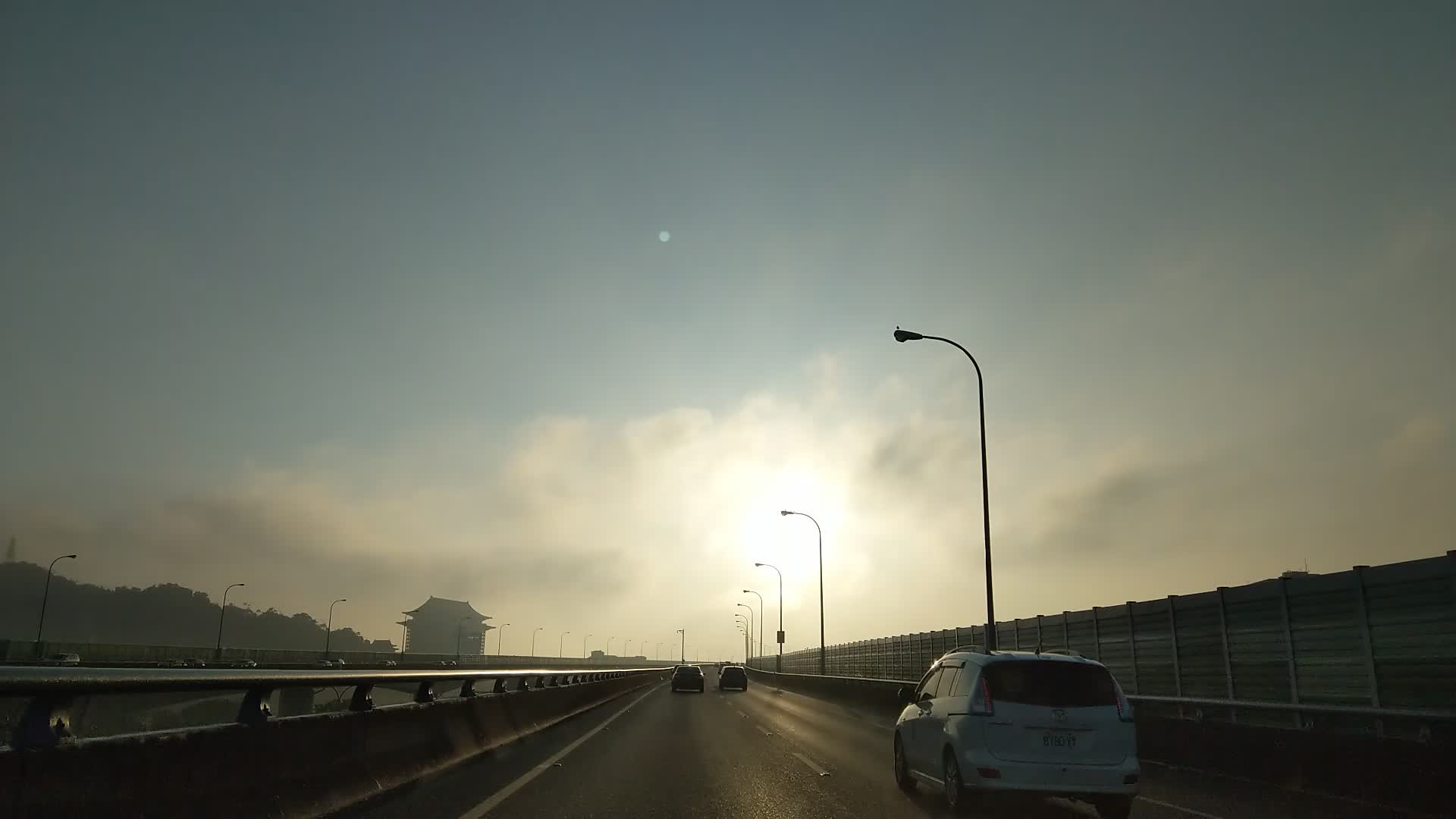The image depicts a horizontal view of a highway scene with moderate traffic flow. A white crossover vehicle can be seen traveling in the right-hand lane, while two darker-colored sedans are positioned ahead, also navigating the highway. The roadway itself appears to be an overpass or bridge, evidenced by the prominent barriers lining its edges. 

In the background on the right, wooden sound barriers obscure the distant horizon, limiting the view beyond. To the left, another two-lane highway for oncoming traffic is faintly visible, marked by numerous street lights, though no vehicles can be seen on this adjacent route at the moment. 

The scene is set against a backdrop of a clear blue sky adorned with scattered clouds, suggesting bright conditions typical of either early morning or late afternoon, hinting at sunrise or sunset. Additionally, some low trees are visible, contributing to the scenic vista. Notably, an impressively sized pagoda with distinct Asian architectural features stands out in the section of the highway designated for oncoming traffic, adding a unique cultural element to the landscape.